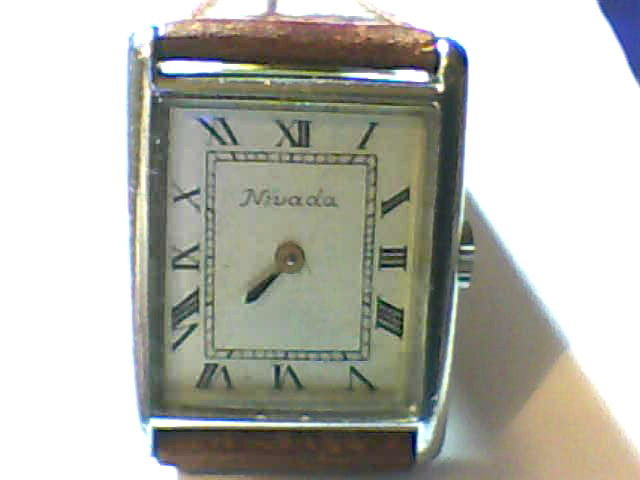This close-up photo captures an antique rectangular wristwatch with a slightly grainy and out-of-focus appearance. The watch features a silver metal body with a rustic charm, and a worn brown leather band connects to the top and bottom, showing signs of age and wear. The winding stem is visible on the side of the watch.

The watch face is white with Roman numerals I through XII arranged in a square layout, encircling an inner square marking that highlights the area where the hands are. Only a single black hour hand is present, pointing slightly past the 7, nearly at the 8. The brand name "N-I-V-A-D-A" is prominently inscribed on the upper part of the face, adding a classic touch to this vintage timepiece.